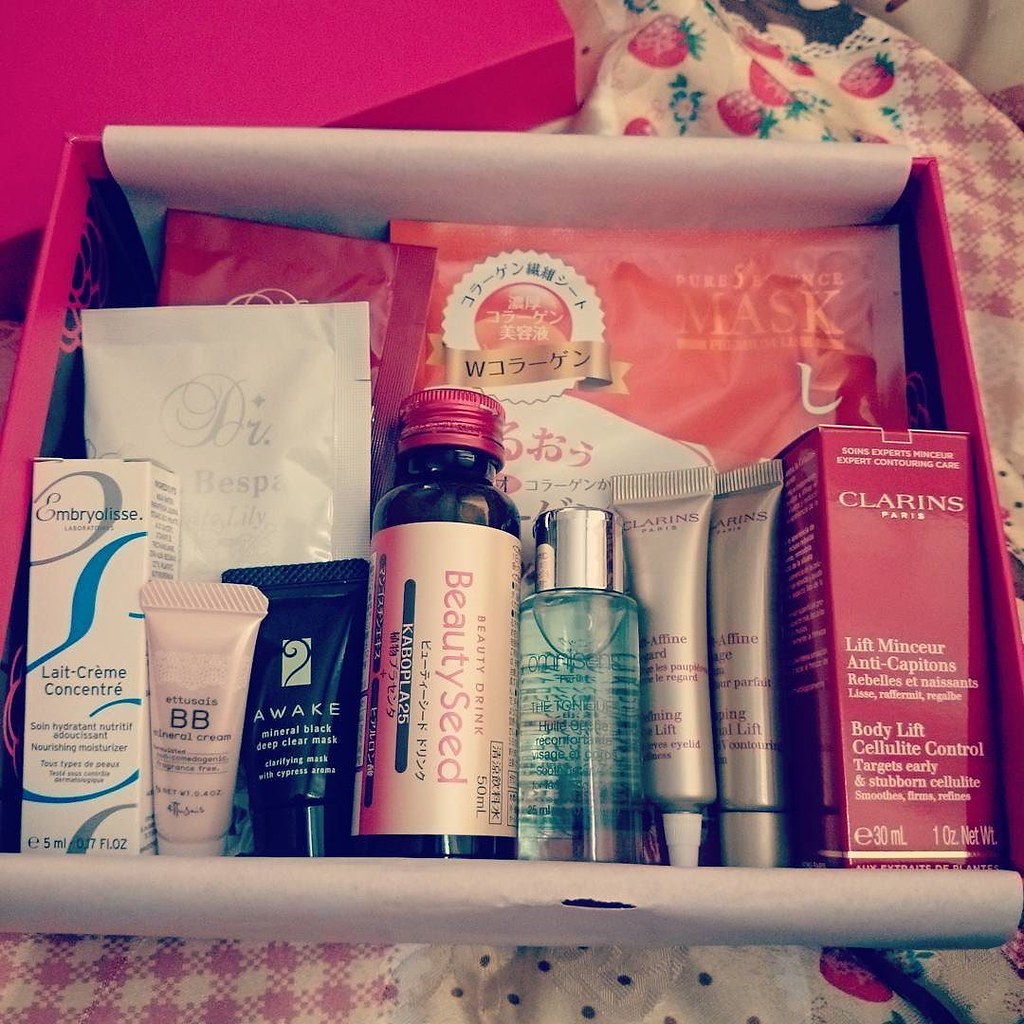This photograph showcases a detailed display of a beauty care box placed on a charming strawberry-patterned cloth, which also features an additional pink and white checkered design. The box itself, made of cardboard, is primarily white with a pink lid, which can be seen resting in the background. Organized neatly within the box are several beauty and skincare products including:

- A burgundy and white plastic package.
- A blue-gray and white box.
- A light pink and white BB cream tube.
- A black product tube.
- A pink-labeled bottle with a pink lid.
- A clear liquid bottle with a silver lid.
- Two silvery tubes, one with a white lid and the other with a silver lid.
- A burgundy-colored box with white lettering that reads "Body Lift Cellulite Control."
- A face mask in a white, gold, and orange packaging tucked beneath the other items.

This curated collection of beauty products suggests a well-thought-out selection of skincare and cosmetic essentials.